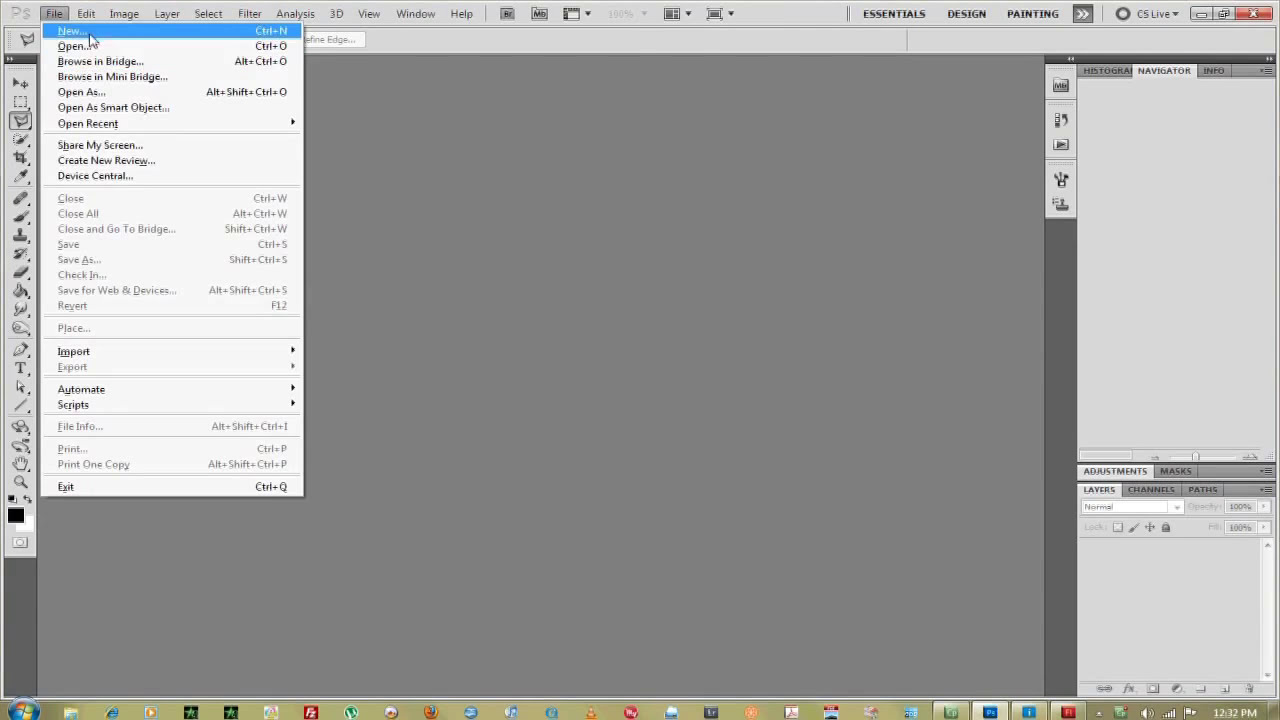This image is a detailed screenshot taken from a Windows computer, likely during the Windows Vista era, indicated by the rounded Start button in the bottom left featuring the colorful Windows logo. The screenshot primarily shows an open application, which appears to be an older version of Adobe Photoshop. The interface includes a gray toolbar on the left side, populated with various graphic editing tools such as brush tools, stamp tools, and text tools. At the top, the file menu is open, with the "New" option highlighted in blue while the rest of the menu is a light white with black text. The main workspace is a large gray rectangle, representing the canvas area, and to the right are additional vertical, lighter gray rectangles that contain more editing tools or options common in graphic editing software. The Windows taskbar at the bottom displays a few icons and the clock in the bottom right corner. The color scheme throughout includes shades of gray, blue, white, and black, with occasional highlights of red, orange, green, and purple.